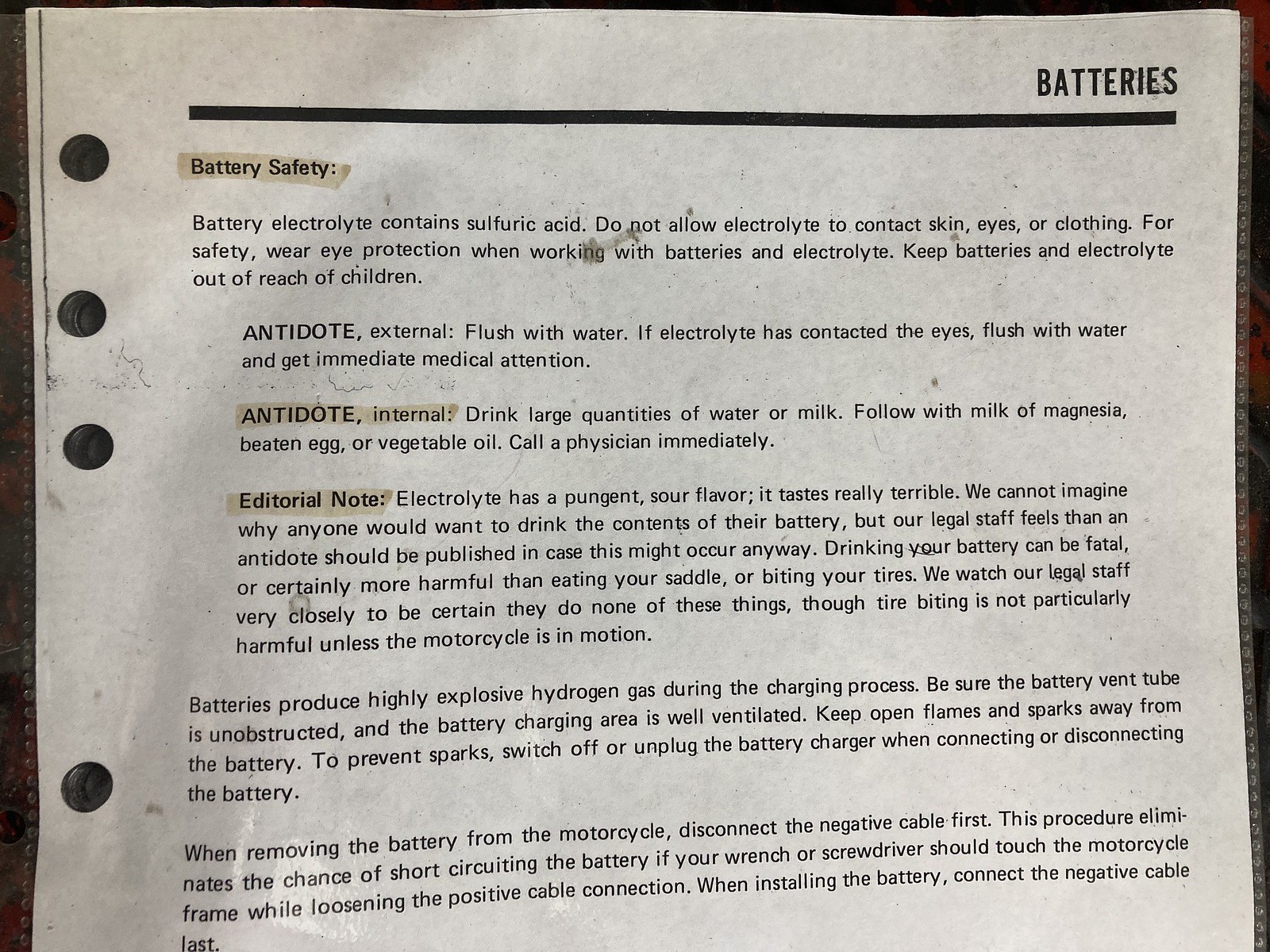This image is a color photograph of the top portion of a printed and possibly photocopied page from a safety manual, which appears to be either laminated or inserted in a plastic sleeve, evidenced by the visible edges of the plastic. Behind the page is a dark background. This slightly dirty and discolored sheet features four punch hole marks down its left side, suggesting it may be designed for inclusion in a binder.

At the top right corner, in bold capital letters, is the word "BATTERIES." Directly below this, a thick black line spans the width of the page, and beneath this line, several paragraphs of text are present. Notably emphasized in faded yellow highlighter are headers such as "BATTERY SAFETY," "ANTIDOTE INTERNAL," and "EDITORIAL NOTE."

The section highlighted as "BATTERY SAFETY" advises that battery electrolyte contains sulfuric acid, which must not contact skin, eyes, or clothing. Safety measures include wearing eye protection and keeping batteries out of children's reach. The "ANTIDOTE EXTERNAL" section instructs to flush the area with water and seek immediate medical attention for eye exposure to the electrolyte. 

"ANTIDOTE INTERNAL" recommends drinking large quantities of water or milk, followed by milk of magnesia, beaten egg, or vegetable oil, and calling a physician immediately. An "EDITORIAL NOTE" humorously indicates that electrolyte has a terrible taste, suggesting it's a highly unlikely material for ingestion but acknowledging the necessity of publishing an antidote. The note adds that batteries produce explosive hydrogen gas during charging, advising proper ventilation and caution to avoid sparks or open flames. Detailed instructions are given on proper procedures for connecting and disconnecting battery cables to prevent short circuits and ensure safety during installation and removal.

Overall, the image documents safety precautions and emergency procedures related to battery handling, framed within a mix of technical and editorial insight, underscoring the importance of adhering to safety guidelines in battery maintenance and use.